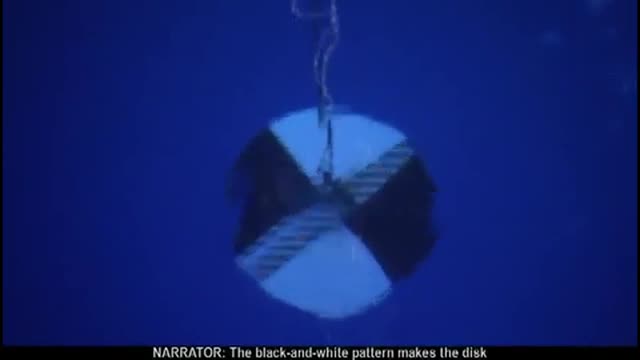In the center of the image, set against a midnight blue background with muted black edges, is a circular object split into four triangular sections, like a pizza. The top and bottom triangles are white, while the left and right triangles are black, creating a striking black-and-white pattern. This object appears suspended by a wire or cable that is partially cut off at the top of the image. The background is dark and somewhat ambiguous; it could be a wall or underwater, contributing to a feeling of distortion. Along a narrow black strip at the bottom, white text reads: "Narrator, the black and white pattern makes the disk."